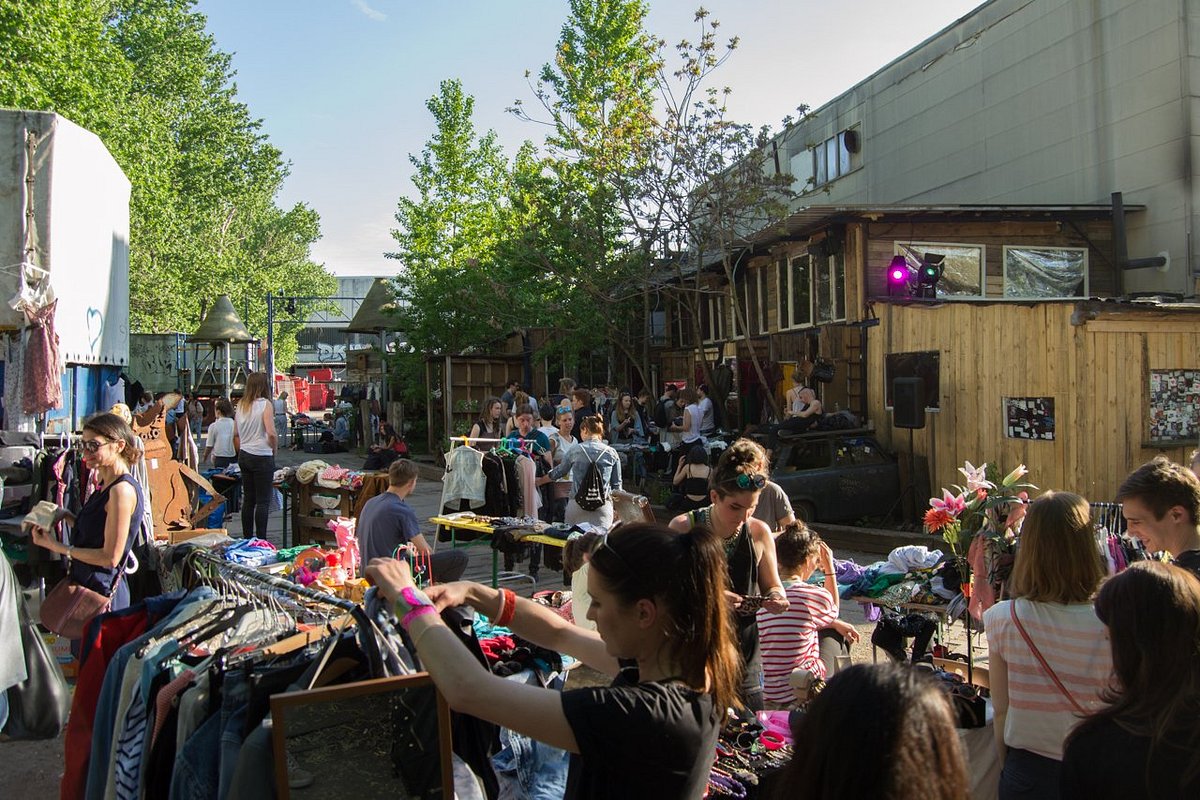The image captures a bustling outdoor market scene set on a city street, likely a flea market or street fair. The area is paved with cement and lined with numerous metal clothing racks and tables overflowing with various garments and jewelry. The racks are prominently filled with clothes on hangers, and tables display an array of jewelry.

In the foreground, to the left, a young woman with brown hair, wearing a grayish-black top, attentively examines a piece of clothing she's holding with both hands from a rack. She appears to be in her early 20s. Nearby, another woman in a white top with yellow and pink stripes has a pink bag slung over her shoulder, while further in the scene, a lady with a black backpack and a white top browses through the racks. 

The market is crowded with people, predominantly women, though a few men are also visible. On the right-hand side of the photo stands a two-story wooden building attached to a taller concrete structure. In front of the gray brick building, there is a smaller shack constructed from brown wooden slats, possibly serving as a DJ booth, complete with tall light stands emitting pink and green lights, and PA speakers set up to provide music.

Further in the background, a young couple stands to the right with the man smiling, both engaged in looking at clothes, while a woman with a child examines a piece of jewelry from a table of accessories. Trees and other urban elements frame the scene, highlighting the vivacious and energetic atmosphere of this community gathering.